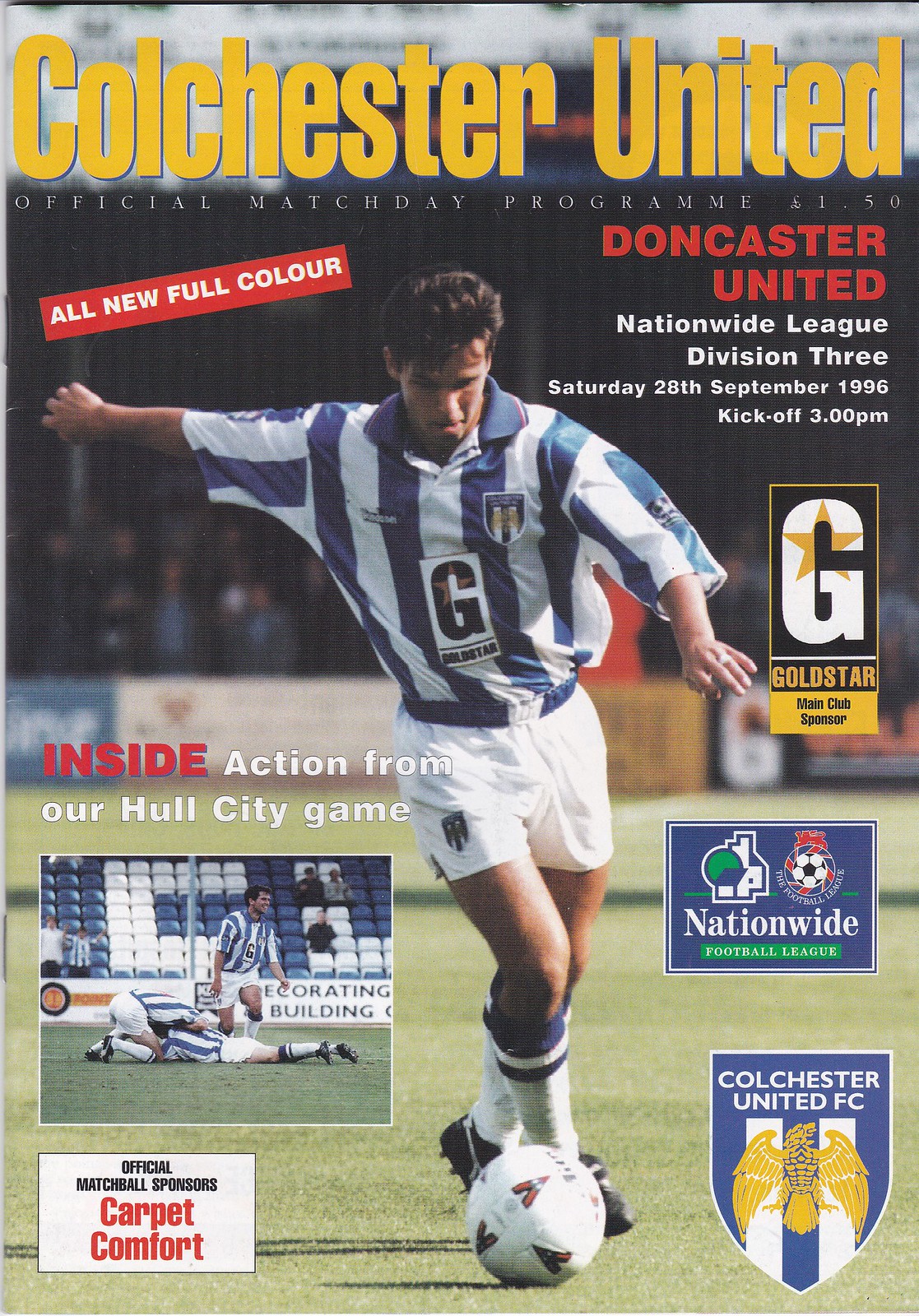This is the cover of a soccer magazine from the UK, featuring Colchester United. Dominating the upper section, the title "COLCHESTER UNITED" is prominently displayed in large yellow letters. Beneath this, on a red background with white text, it reads "OFFICIAL MATCH DAY PROGRAM EURO 1.50" and further comprises "DONCASTER UNITED" in red. The magazine details are laid out clearly: "Nationwide League Division 3, Saturday 28th September 1996, Kickoff 3.00PM."

The focal point of the cover, set against the backdrop of a sports field, is a photograph of a soccer player poised to kick a football lying on the grass. Dressed in a blue and white jersey adorned with a black "G," white shorts, blue and white striped socks, and black shoes, the player's right arm is extended backwards while his left hand points towards the ground. 

To the left of the main image, a smaller rectangular photo captures some players and a referee on the ground, accompanied by the text "INSIDE ACTION FROM OUR HULL CITY GAME," with "INSIDE" highlighted in red. The lower section features logos from various clubs and companies, such as Nationwide and Colchester United, enhancing the visual and informational richness of the cover. An advertisement for "Carpet Comfort" is also present.